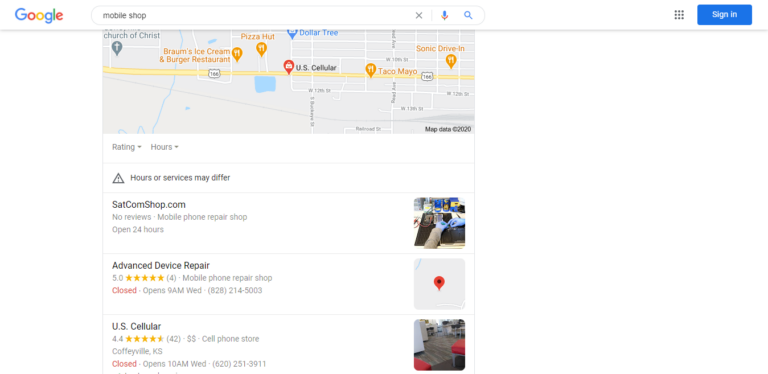A bustling cityscape featuring a variety of colorful storefronts and signs indicative of a typical commercial district in Los Angeles. Prominent among these are fast-food giants like Taco Bell, Sonic Drive-In, and Pizza Hut, each vying for attention with vibrant neon lights. Not far away, a Dollar Tree store adds to the array of retail options available to residents and visitors alike.

In the foreground, a vintage mobile shop adorned with a sign reading "Open 24 Hours" showcases its eclectic range of merchandise through its windows. This shop seems particularly well-rated, boasting five gold stars from 42 reviews and an impressive 4.4-star rating for another cell phone store. An overhead sign mentions U.S. Cellular and indicates operating hours starting from 9 a.m. on Wednesday.

Digitally overlaid on the image is a navigation interface showing map data, a magnifying glass indicating search functionality, and options to sign in. A close-up portion of the digital map mentions corporate information and probable turn-off times. Below this, phone numbers for various businesses are listed, suggesting comprehensive local business details.

A Panda Express is subtly featured next to a restaurant offering familiar fast-food fare. Mixed in among these are a microphone icon and miscellaneous labels hinting at diverse businesses ranging from furniture stores to ice cream parlors scattered throughout the frame. The dense, sign-laden image encapsulates the lively spirit of urban commerce, all set against the broader backdrop of the city of L.A.